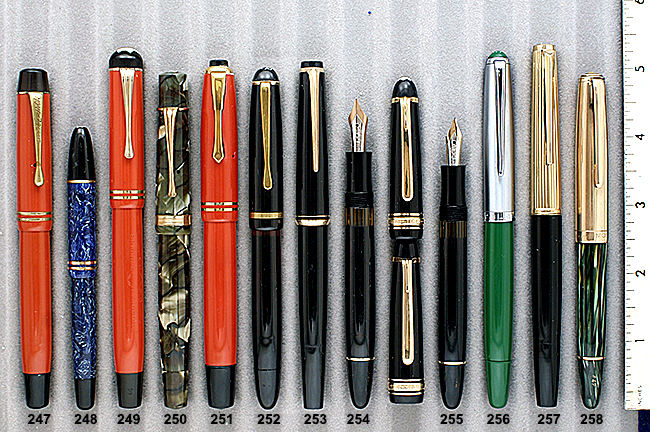This image features a detailed arrangement of 13 fountain pens and ballpoint pens, sequentially organized from left to right and aligned vertically against an off-white and tan striped background with grooves designed to hold the pens' contours. The pens are evenly spaced and positioned alongside a ruler on the right-hand side, allowing precise measurement of their lengths. Each pen is labeled with a three-digit number ranging from 247 to 258, though one pen lacks a number. The collection showcases a variety of colors and trims: red, blue (some with marble patterns), gold, black, and green. Several pens feature either gold or silver ends. Specifically, the red and black pens are prominent, some of which display their nibs due to the missing caps. This meticulous arrangement offers a clear and comprehensive view of the pens' distinct designs and lengths.